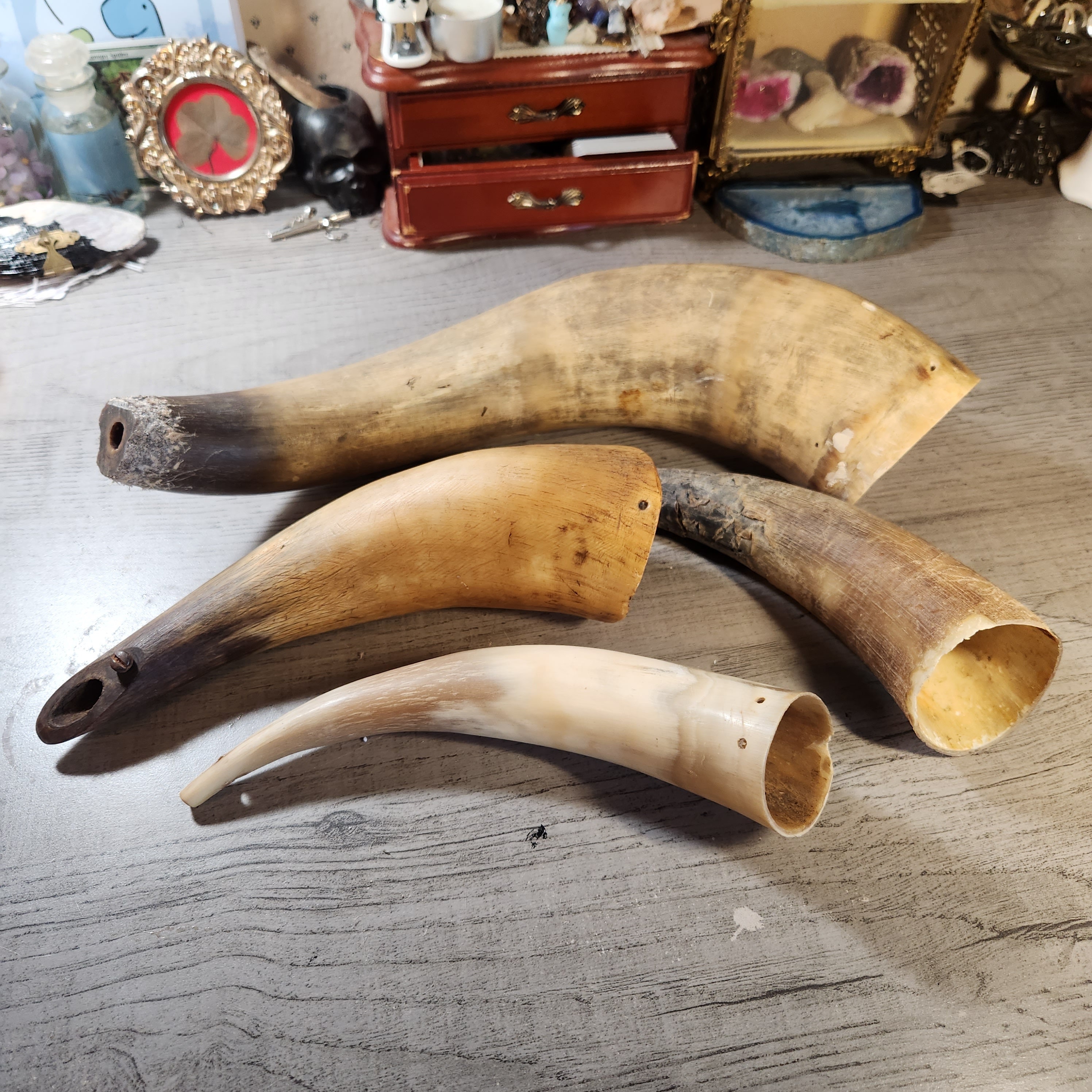In this photograph, four slightly curved horns, varying in size and shape, are placed on a wooden surface. The horns, primarily brown but with some showing tan, white, or blackened tips, appear empty and hollow, likely animal in origin. They range from sharp to blunt and the largest is about three times thicker than the smallest. Surrounding these horns, the wooden table holds an eclectic assortment of old items. In the background, decorative trinkets, including small rocks, a black jar, tiny bottles, and a small brown cabinet or drawer, suggest an antique collection possibly arranged in an attic-like area.